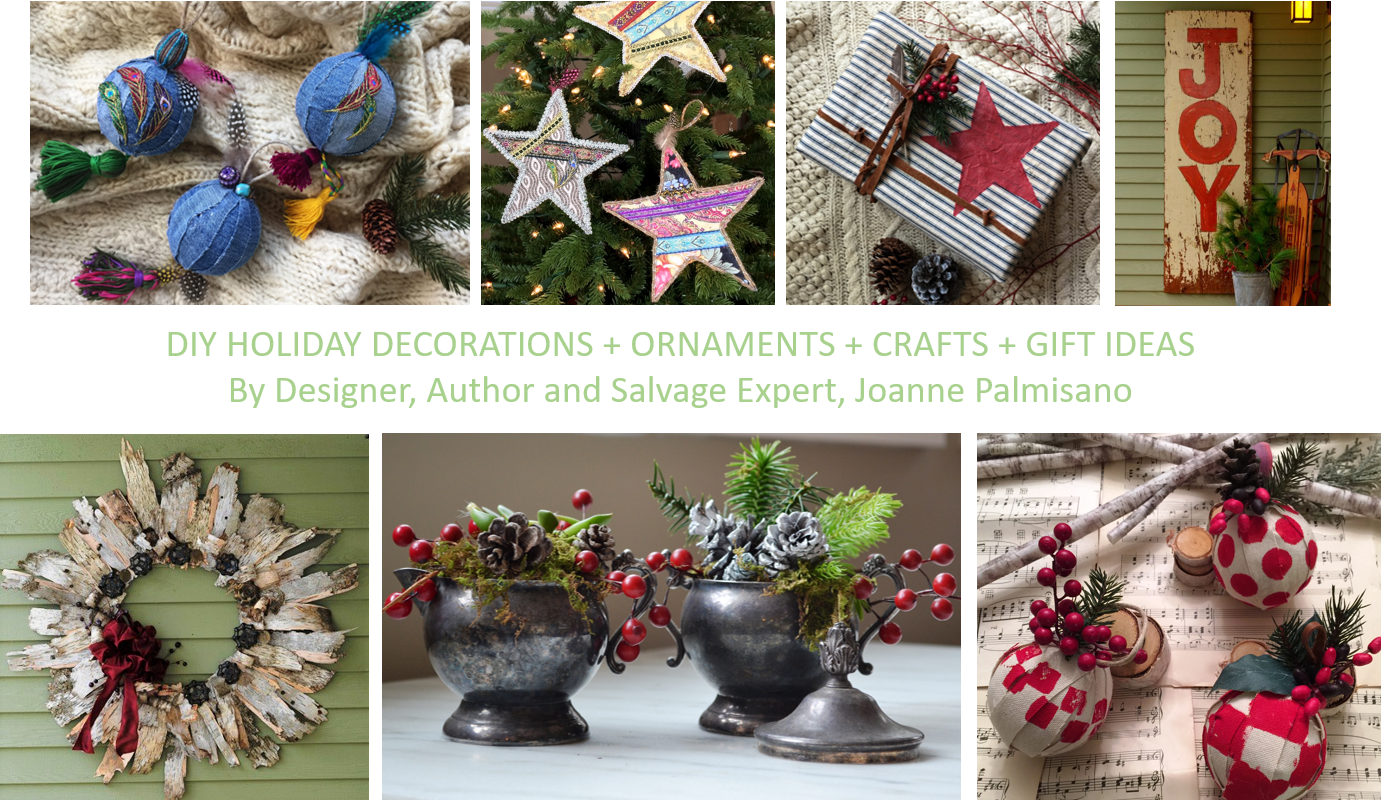This image is a collage of DIY holiday decoration ideas, featuring a central caption in green text on a white background that reads: "DIY Holiday Decorations + Ornaments + Crafts + Gift Ideas" by designer, author, and salvage expert Joanne Palmisiano. The collage consists of seven smaller photographs. 

At the top left, three round ball ornaments wrapped in denim fabric adorned with peacock feather designs rest on a white blanket. The top middle image showcases three custom star ornaments illuminated by lights on a green Christmas tree, featuring a variety of colors like purple, pink, white, blue, red, yellow, gray, and black. To the top right, we see a small red star on a gray and white striped gift box wrapped with brown straps.

The image directly to the right of the text features a rustic "JOY" sign in red letters on a piece of brown wood next to a brown wooden sleigh. This scene is decorated with a small green plant in a white or tin silver flower pot illuminated by a yellow light from the top right.

On the bottom left, a green house's siding serves as a backdrop for a white waxed wreath adorned with a red ribbon. The middle bottom image displays two silver tin containers with green leaves, mistletoe, and brown pinecones arranged on a white table against a tan wall. Lastly, the bottom right picture features three red and white ball ornaments with holly designs, set against a backdrop of white sticks with gray accents and black and white music note decorations.

Overall, the collage incorporates various holiday themes with vibrant colors like red, green, and blue, featuring assorted ornaments, wreaths, gift ideas, and festive decor.